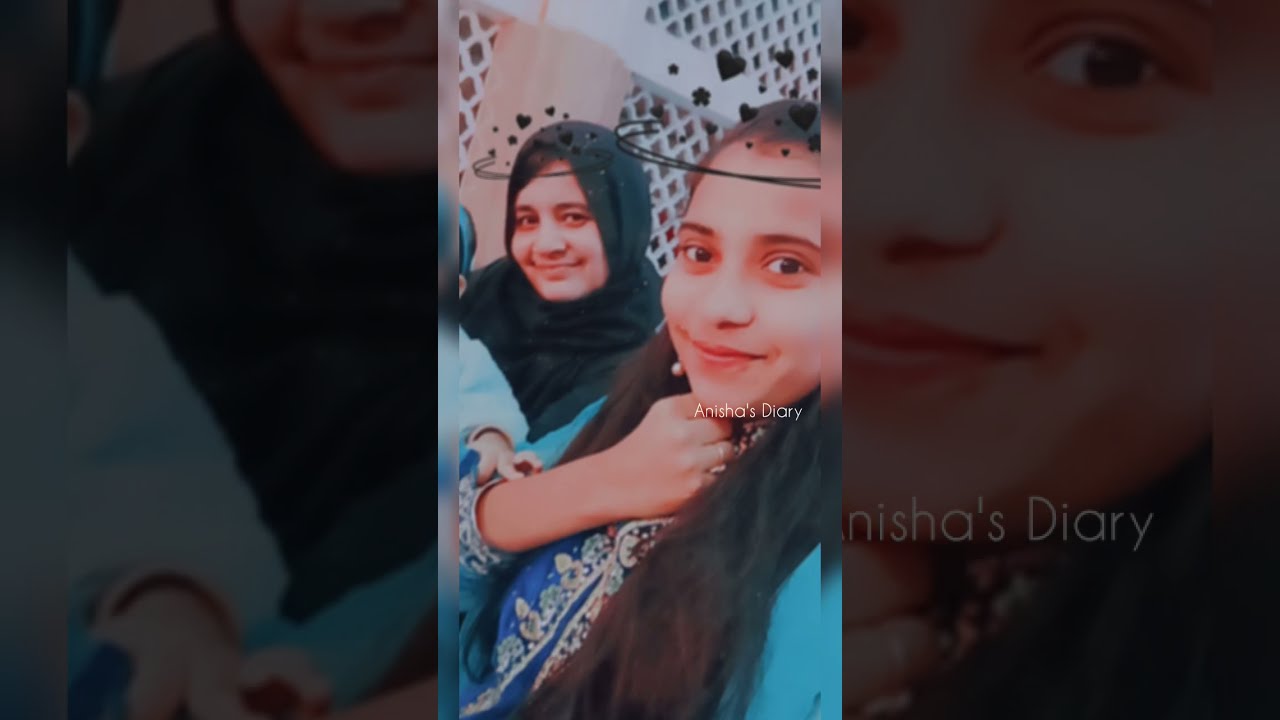The image is a horizontal rectangular screen capture featuring a vertical video centered between echoed, zoomed versions on both sides with wide, dark borders. The central photograph is of two women, possibly a young woman or else a mother and daughter, dressed in traditional attire. The woman in the background wears a blue dress and a black headscarf, smiling subtly with her mouth closed, while a child seems to be on her lap. The woman in the foreground has long black and brown hair, wears a blue sari with a scarf around her neck, and is smiling pleasantly with her right hand clasped under her chin. Both women appear happy, and above their heads, there are black graphic overlays featuring hearts and stars, giving the impression of face filters. They are standing outside in front of a peach and white building with crisscross accents. The text “Anisha's Diary” is centered at the bottom of the image.